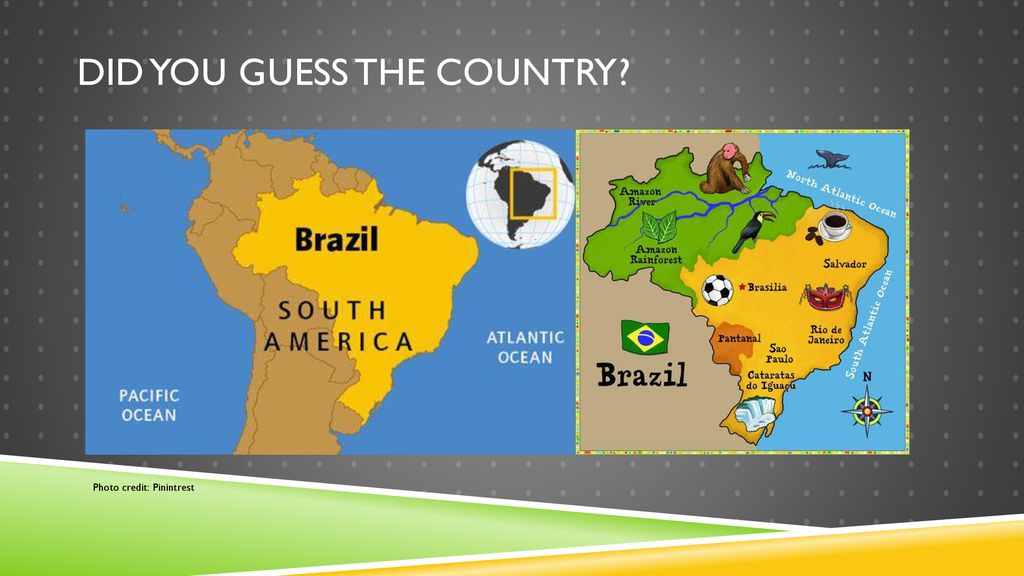The image is a detailed screenshot featuring a gradient background that transitions from dark gray on the left and right edges to light gray in the center. Overlaid in white text at the top, it asks, "Did you guess the country?" The map prominently displays South America, with Brazil highlighted in yellow and the rest of the continent in brown. The geographical focus includes both the Pacific and Atlantic Oceans.

Accompanying the map, a globe features a highlighted yellow rectangle, zooming in on the area depicted. To the right of the map, Brazil's green flag with a yellow diamond and a blue circle is prominently shown. Major geographical and cultural landmarks within Brazil are marked, including the Amazon River, Amazon Rainforest, Salvador, Brasilia (indicated with a red asterisk), Rio de Janeiro, São Paulo, and the "Cataratas do Iguaçu" (Iguaçu Falls).

Both the North and South Atlantic Oceans are labeled, and a compass is present along with decorative yellow and green triangles at the bottom of the image. The photo credit at the bottom right corner attributes the source of the image to Pinterest.